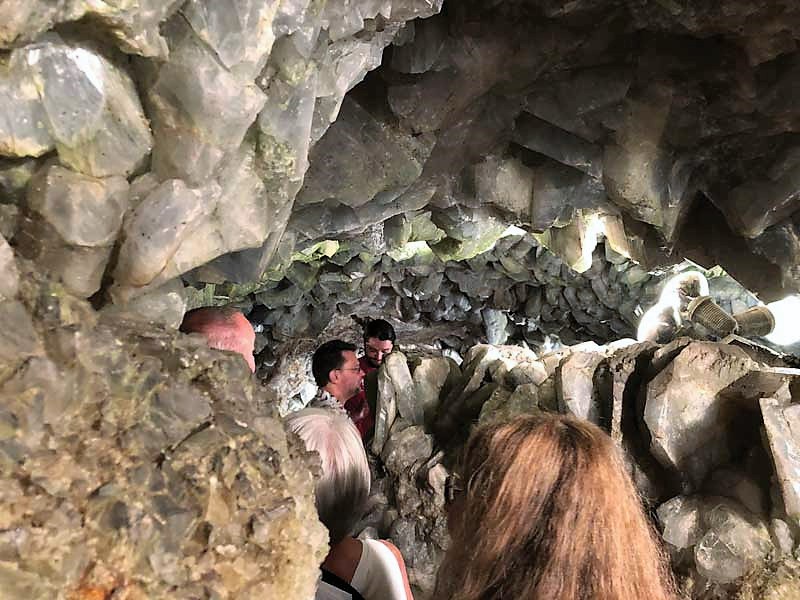In the narrow, dimly-lit quartz-filled cave, five people navigate a winding path through the towering, shimmering rock formations. Two men in their 40s, a woman in her 40s, and a couple in their late 60s weave through the cave's intricate layout, their heads occasionally obscured by large quartz columns. The cave ceiling is low, just two to three feet above the tallest heads, adding to the sense of adventure. The quartz varies in color, from dark charcoal and brown to the more familiar white and clear crystals, with occasional greenish hues. Two lamps illuminate this underground spectacle, casting light on the rich mineral surfaces and ensuring the path is visible. The image prominently features the backs of a blonde-haired woman and a white-haired woman, suggesting perhaps a guided tour. In the immediate foreground, next to a large rock column, an opening hints at a possible exit or just another section of the cavern yet to be explored.